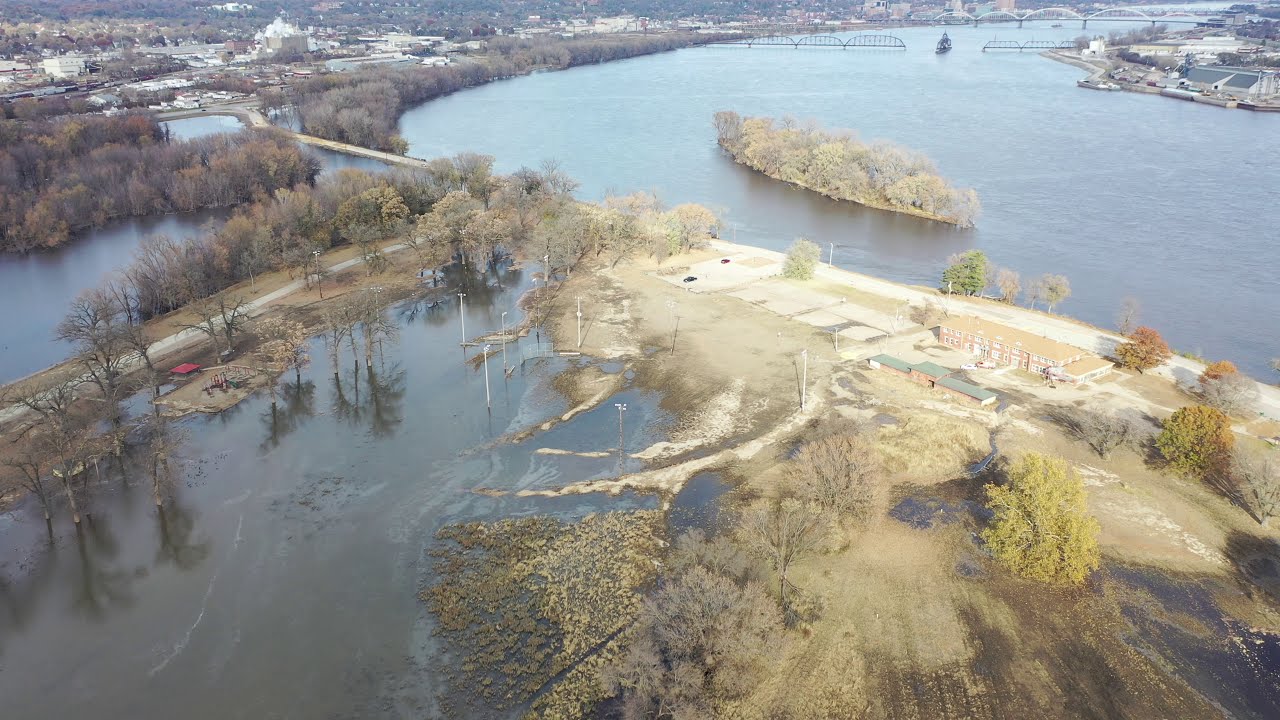This aerial photograph features a complex scene centered around a major river and depicting flood damage. In the foreground, where the levee has clearly broken, you can see significant flood damage on the south side of the image. Nearby, the busted levee was meant to contain a large river that now appears murky and swollen. Adjacent to the levee break, a road is closed off with a blockade, and no cars are visible, signifying restricted access due to flooding. 

Further into the background, a sizable bridge stretches across the river but is notably damaged, with a section that has collapsed. This bridge originally connected a predominantly residential town on the left, featuring many houses, and an industrial area on the right, comprising warehouses and office buildings.

To the right of the image, swampland bordered by brown trees and bushes enclose another large body of water. In the center of the water stands a bridge that also connects to a sandy, possibly recently renovated or constructed, island-like structure. This island area appears to consist of white and gray dirt, without visible construction equipment but suggesting recent activity. Surrounding the closed road are trees lining the way.

Above, the sky is overcast with hints of sunlight breaking through, presenting a partly sunny but mostly cloudy day. Off in the distance, the bridge appears to function as a drawbridge, as evidenced by a boat navigating between its opened sections. The overall scene captures a moment of natural disruption mingled with human infrastructure, depicting both the tranquil prelude and the chaotic aftermath of a flood.